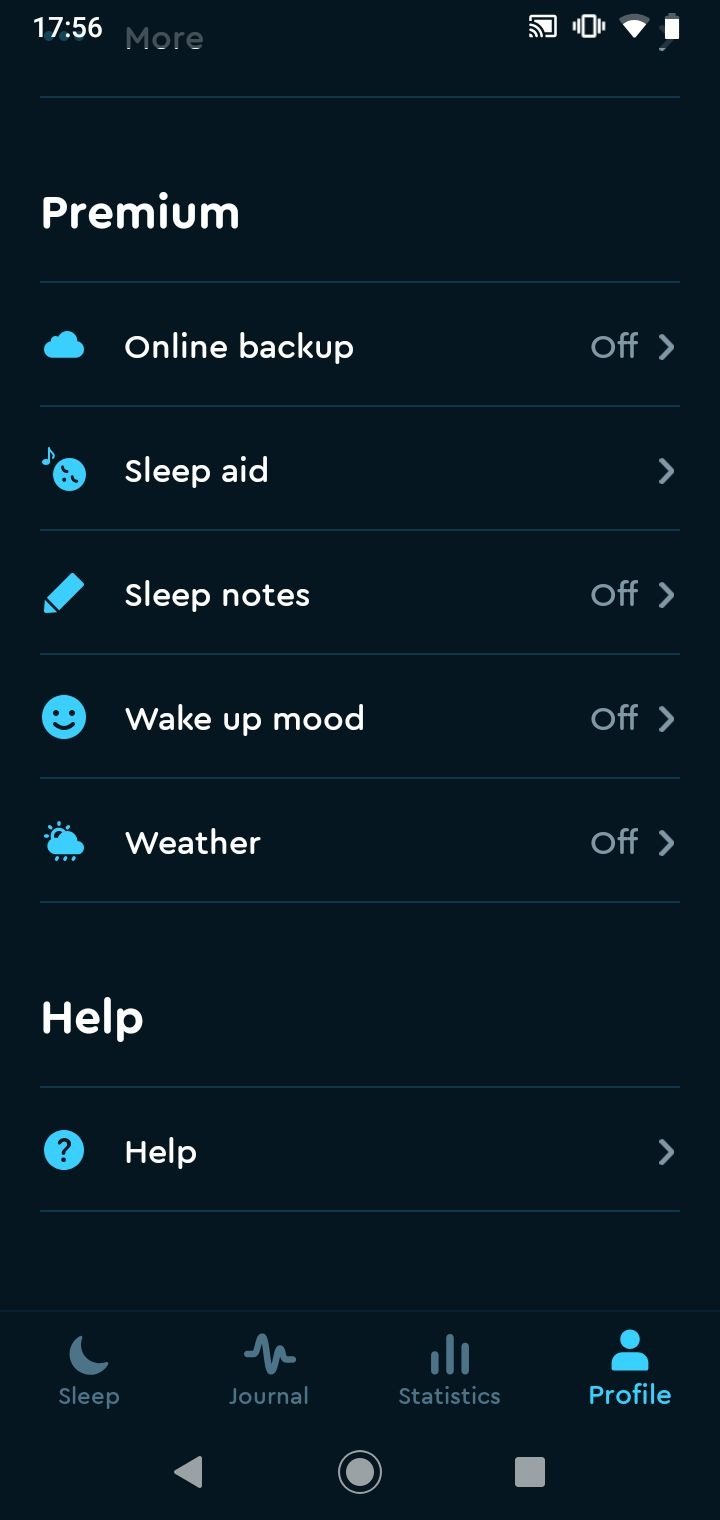On the screen, the time is prominently displayed as "17:56" at the top, accompanied by various status icons including cast, vibration mode, Wi-Fi connection, and battery life indicators. Below this, a notification states "Premium Online Backup: Off," next to a blue cloud icon. The interface also features a "Sleep Aid" section represented by an arrow pointing to a silhouette of a cartoon character's head, seemingly sleeping with music symbols around it. The settings for "Sleep Notes," "Wake Up Mood," and "Weather" are each marked as "Off," with corresponding icons: a blue pencil, a blue smiley face, and a blue cloud with sun and rain, respectively. A "Help" section is indicated by a blue circle with a question mark and an arrow. The screen displays menu options such as "Sleep" set to "Normal," "Statistics," and "Profile," with the "Profile" option highlighted in blue. Navigation elements include a back arrow, a home button, and tabs for additional functionality.